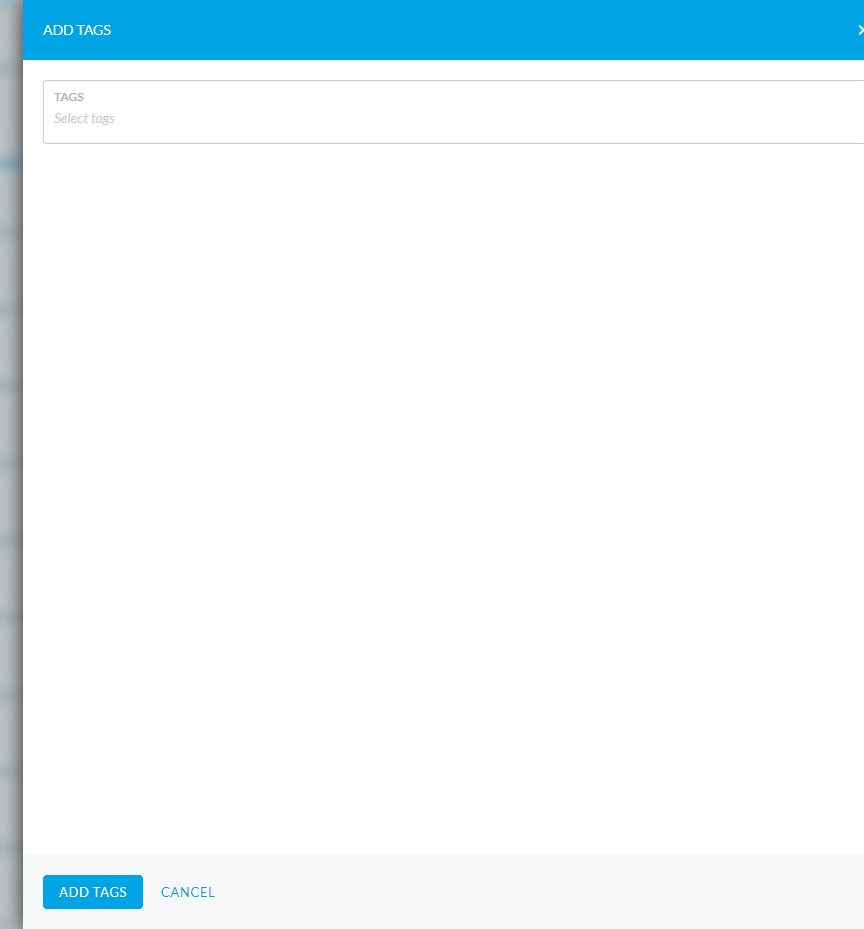A screenshot of a minimalist web page is depicted, featuring a predominantly blank, white interface with minimal elements. At the top of the page is a solid blue banner, within which is situated white text in the upper left corner stating “Add Tags.” Below this banner, the page is largely empty, creating an expanse of white space that invites further content which yet remains undisplayed. 

Approximately centered within this white void is a single gray text box with placeholder gray text that reads, “Select tags.” This text box is currently empty, indicating no tags have been chosen. Beneath the text box, the white space resumes, possibly intended as a placeholder for a list of selected tags, which here is notably absent. 

At the very bottom of the page, a blue button with white text boldly declares, “Add Tags.” Adjacent to this button, a blue text link offers the option to “Cancel,” providing a subtle but necessary action alternative.

Overall, the web page exudes simplicity with its bare-bones aesthetic and the potential for interactive elements centered around tagging functionality, though currently devoid of any user input or tags.